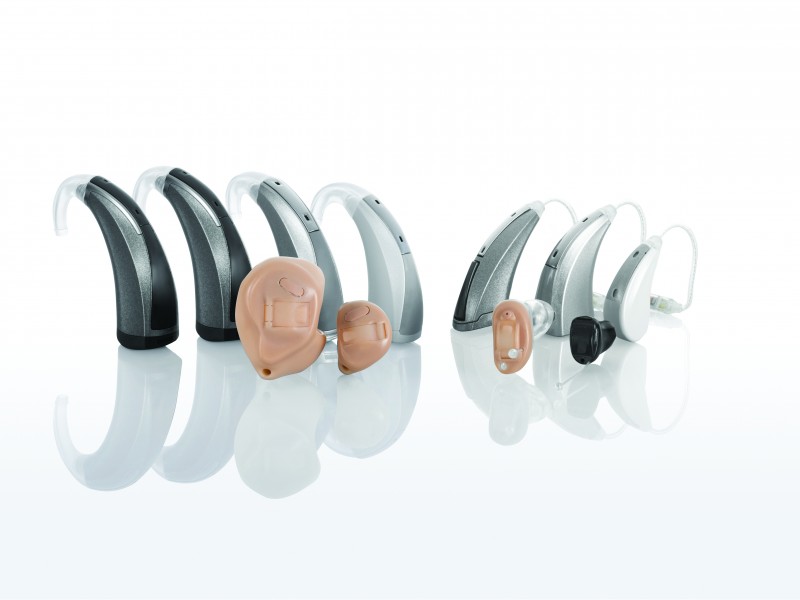This promotional photo showcases a close-up array of modern hearing aids set against a pristine white backdrop. Arranged on a reflective white glass tabletop, these devices are presented in a visually appealing manner, emphasizing their sleek and contemporary designs. The composition includes seven behind-the-ear hearing aids, predominantly in dark black, gray, and silver hues with distinctive white cords that loop elegantly over the ears. Additionally, there are four in-ear hearing aid inserts displayed in front, with three in flesh tones and one in black, all meticulously aligned to help potential users envision the fit and functionality. The reflective surface beneath creates a subtle mirror effect, enhancing the overall aesthetic of this artistically rendered promotional image.